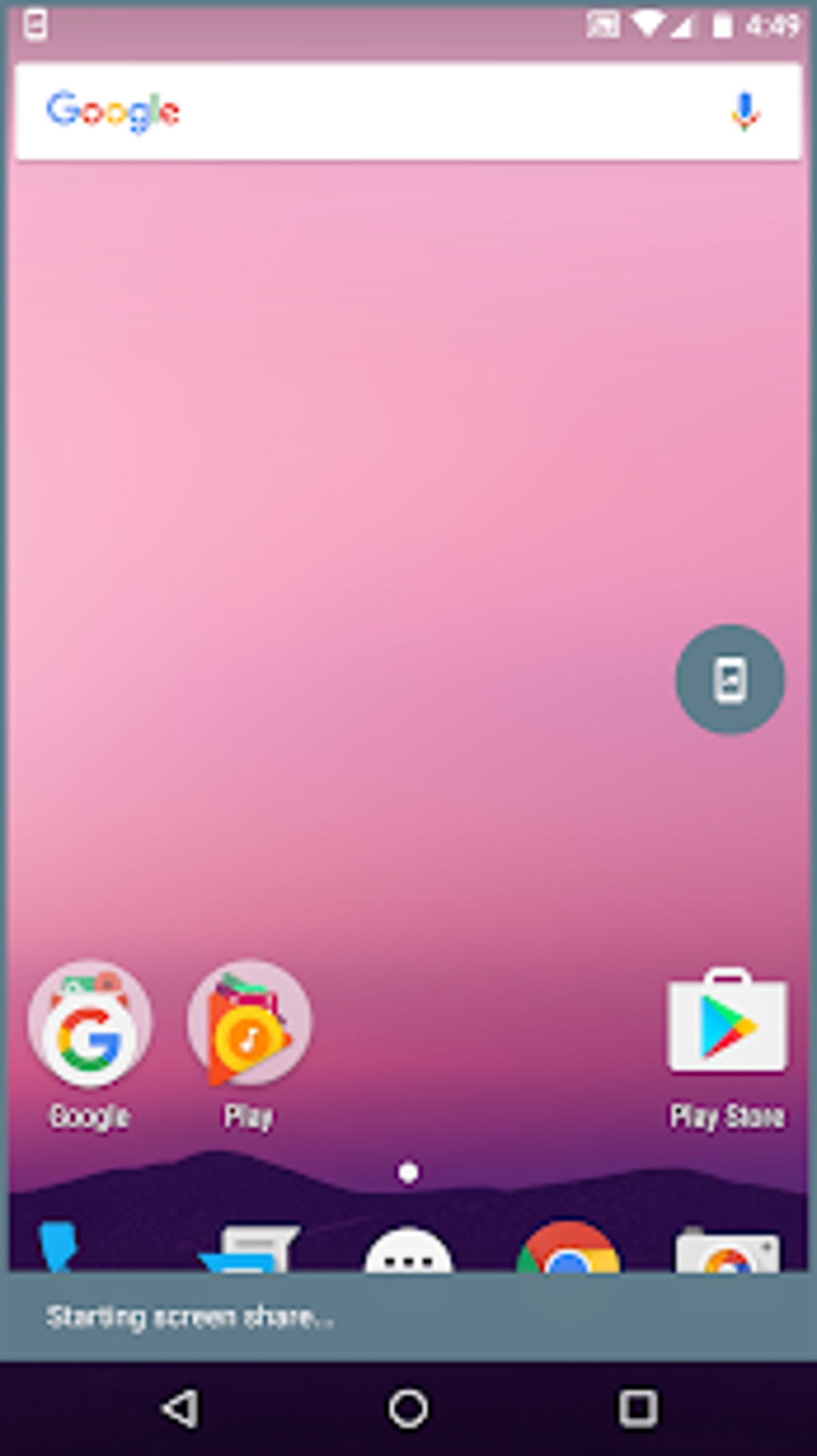The image displays an iPhone screen with a battery level of 44% indicated in the top right corner next to a white battery icon. Dominating the top section is the Google search bar, featuring the word "Google" on the left and a blue microphone icon on the right. The background of the screen transitions from a pink shade at the top to a purple hue at the bottom.

Beneath the search bar, there is a gray circle containing a white cell phone icon. Directly below this circle, there is a white square with the tip of an arrow inside, rendered in blue, red, and yellow colors. Below this icon, in white text, it reads "Play Store."

To the left of this square, there is an orange rectangle containing an orange circle, with the word "Play" written in white below. Further to the left, another circle features the letter "G" in Google's signature colors: red, yellow, green, and blue. Below this circle, the word "Google" is printed.

Lower on the screen, a long gray rectangle with the text "Starting Screen Share" is visible. Finally, at the very bottom of the screen, there is a black line with a white circle in the center, representing the Home button.